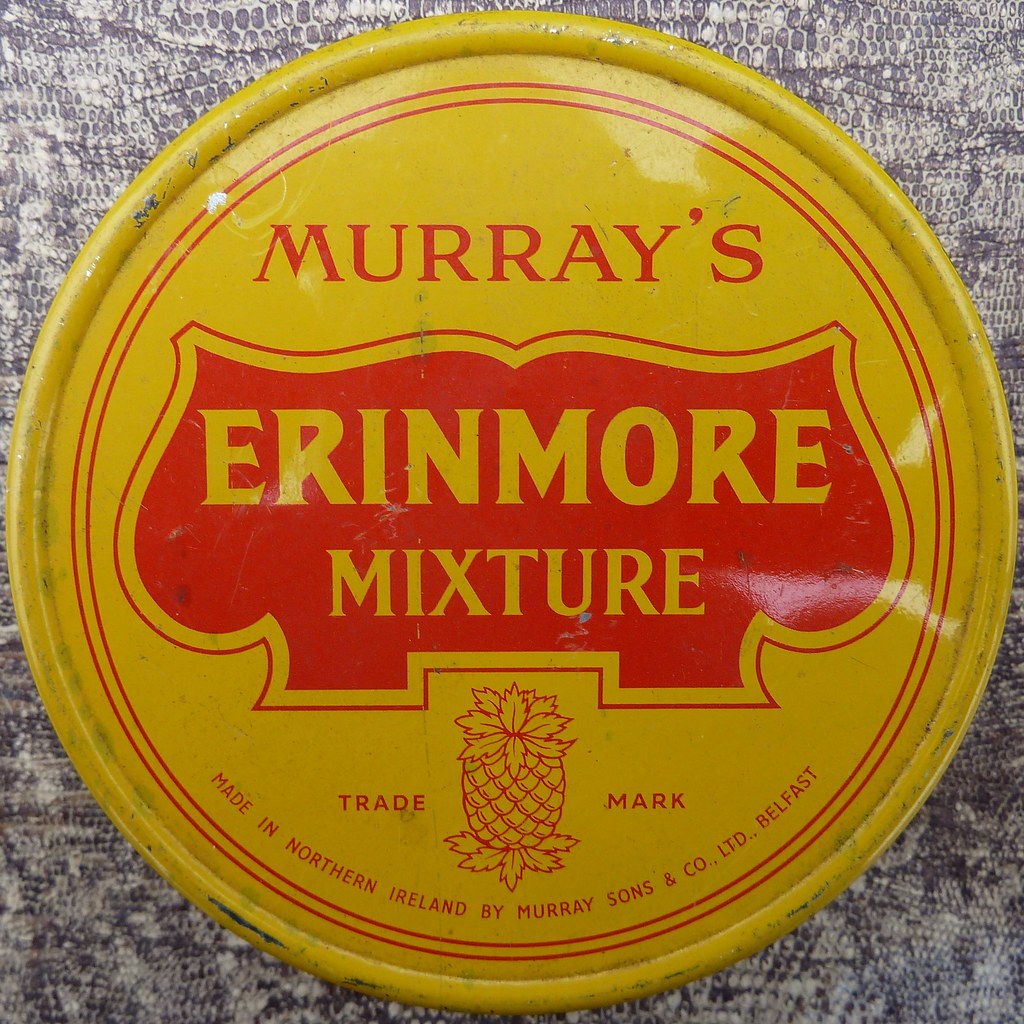This detailed photograph showcases a circular metallic bottle cap, prominently positioned in the center of the image against a soft, textured fabric surface that features a gray and white snakeskin print. The cap itself is yellow, with an outer raised ring. Encircling the inner part of the raised ring are two red pinstripes. At the top center of the cap, in red text, the word "Murray's" is clearly marked. Below this, there is a design resembling an open book on a footed table, with a red background featuring the inscription "Arrynmore Mixture" in yellow print. Further below, a red illustration of a pineapple is flanked by the words "trade" on the left and "mark" on the right. Curving along the bottom edge, from approximately the seven o'clock to the five o'clock position, the text reads "Made in Northern Ireland by Murray Sons & Co Ltd Belfast," also in red. The image is taken indoors with a close-up focus, emphasizing the intricate details of the bottle cap’s design and the fabric’s pattern.